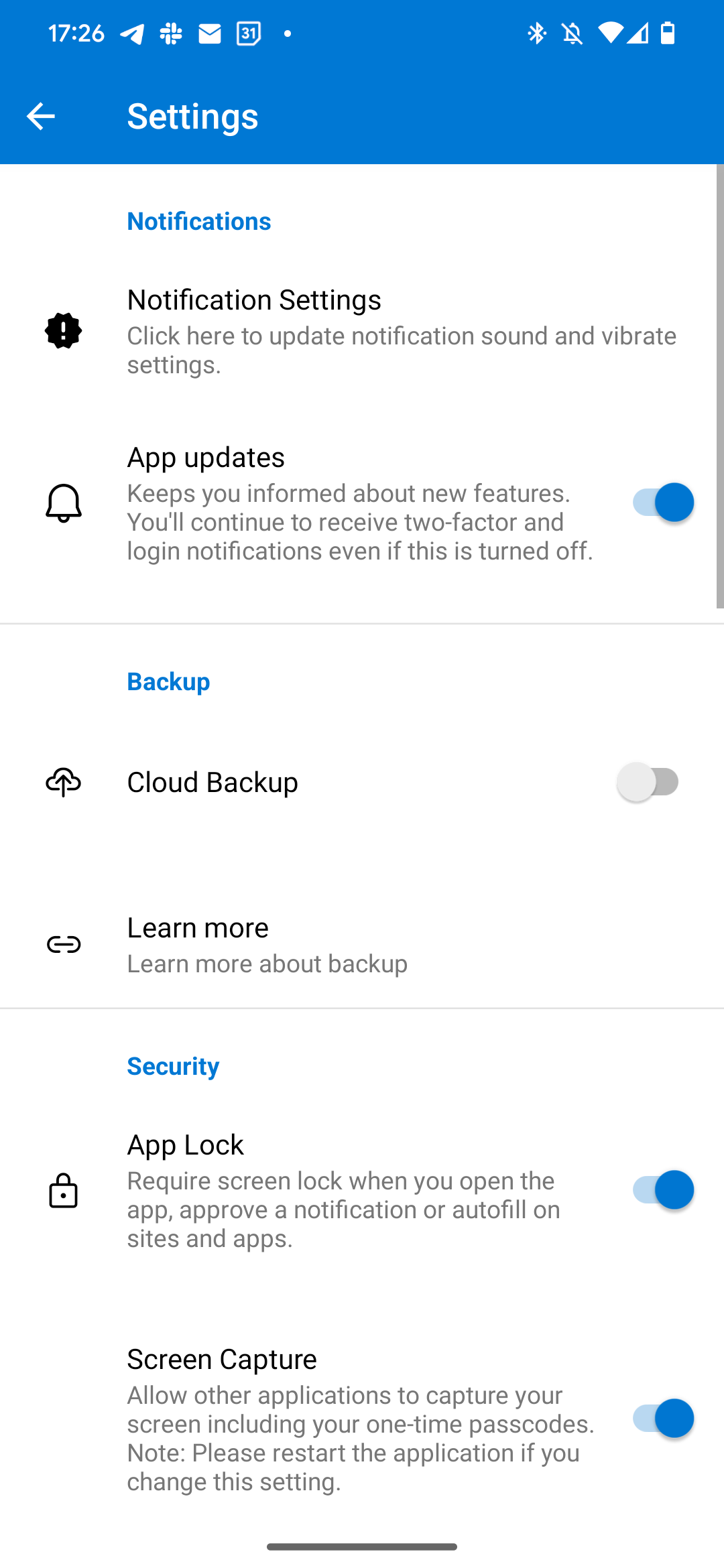A detailed screenshot of a cell phone's settings menu is displayed. At the top, a blue bar shows military time as 17:26, equivalent to 5:26 PM. The screen has a white background with a nearly full battery, active Bluetooth, and strong internet connection. No notifications are visible.

The settings menu is open, with various options listed in blue text. The first section labeled "Notifications" features a gear icon with exclamation points, indicating settings for updating notification sounds and vibration. Nearby, a bell icon signifies app update settings, which are currently enabled.

Below, the "Backup" section, marked with a blue title, includes options for cloud backup, featuring a cloud logo on the left. This backup feature is currently disabled, with an option to learn more about it.

The final section, "Security," involves app lock settings requiring screen lock for app access. This ensures the phone is protected. Additionally, screen capture settings, which allow other apps to capture the screen, including one-time passcodes, are enabled. A note advises restarting the application if this setting is changed.